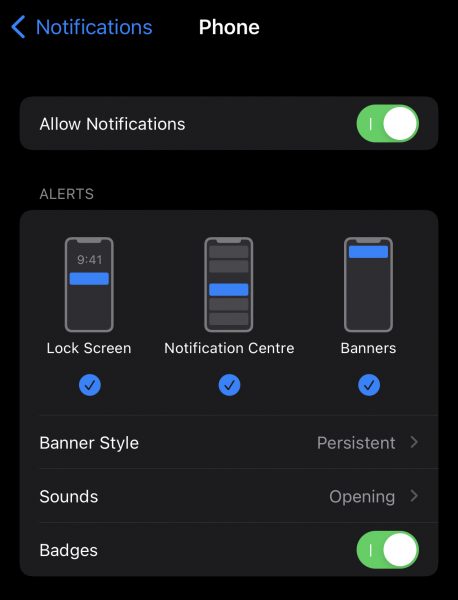The image appears to be a screenshot from a phone’s notification settings menu, set against a black background. At the top center in large white letters is the word “Phone.” In the upper left corner, there is a blue back arrow, and to its right, in blue text, it says “Notifications.” Below that, on the left side in white text, it says “Allow Notifications,” with an oval green toggle button next to it on the right, currently switched on, displaying a large white circle. Below this section, in a lighter white font, it says “Alerts.”

The next section features a horizontal layout of three different cell phone mockups, each outlined in gray. The phone on the left shows a gray time of "9:41" with a green and white bar indicating "Lock Screen" beneath it. The center phone has two gray bars at the top, a blue bar in the middle that says "Notification Center," and two more gray bars at the bottom. The phone on the right shows a blue bar at the top with the rest in black, labeled "Banners" in white text. Each of these three phone mockups has a blue circle with a black check mark below them, denoting selection.

At the bottom of the image, there are more setting options. On the left, it says "Banner Style" in white, and on the right, it specifies "Persistent." Below that, in white text, it says "Sounds," and on the right, it says "Opening." The final entry is "Badges" in white, with an oval green toggle button to the right that is switched on, displaying a large white circle on the right.

This detailed overview reflects the various customization options available for the phone's notification settings.